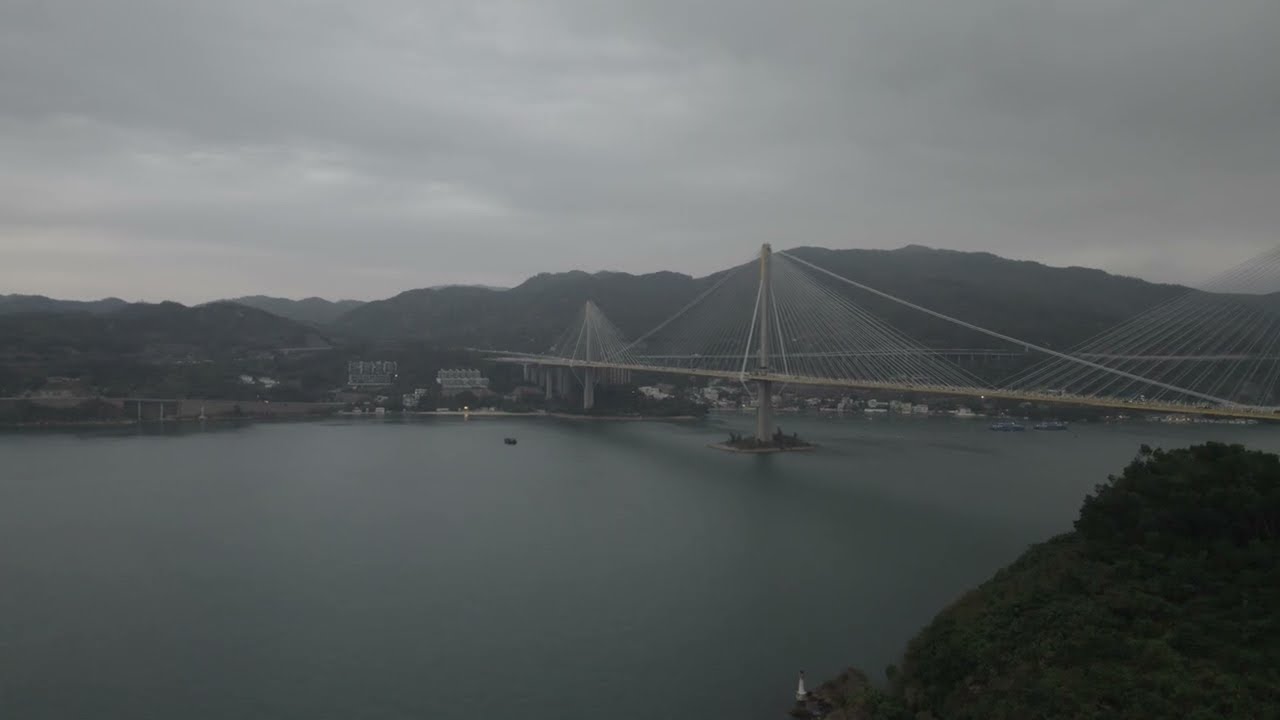The image depicts a large structural bridge spanning across a wide body of water, viewed from a cliffside vantage point. The bridge, central to the composition, stretches from the foreground to the opposite side of the water where it connects with hilly or mountainous terrain. Supporting the bridge are concrete masts and beams, with a network of cables descending on both sides. The weather appears overcast and possibly rainy, casting a dark and dreary atmosphere with a sky full of dense clouds.

The area under the bridge includes an island holding one of the concrete masts, and smaller boats are visible on the water, including a prominent small black boat near the center left. Larger boats and a port or city cluster along the river's edge in the background to the right of the bridge. The landscape beyond the river showcases more hills extending into the distance. In the foreground, the cliffside is covered in vegetation, marking the immediate edge over the water. Sparse buildings on the opposite shore add to the scene, which is devoid of any visible people, underscoring the bleak weather conditions.